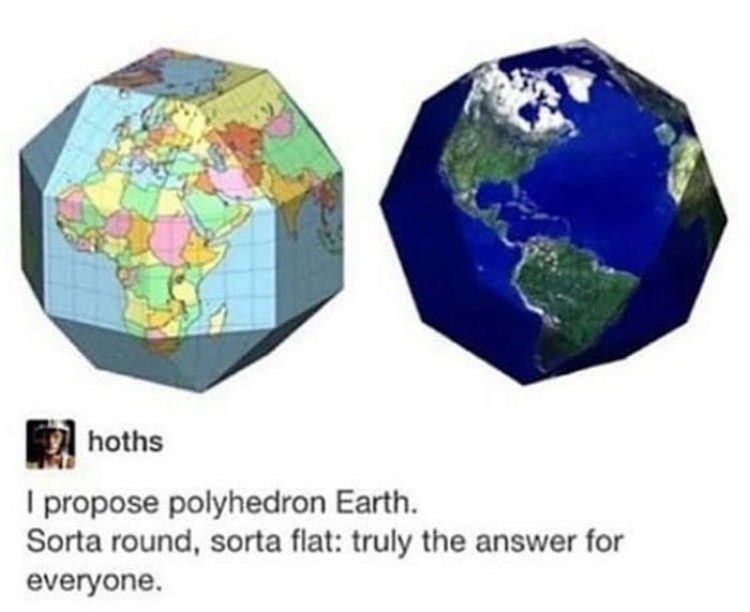In the image, there are two detailed illustrations of Earth depicted as polyhedrons. On the left side, the polyhedron Earth has a light blue background, showing various countries in different colors with visible grid lines, highlighting continents like Africa and Asia as seen in an atlas. On the right side, the polyhedron Earth features a dark blue sea with noticeable green and white continents transitioning from South America to North America, with the northern regions like Greenland and Canada appearing completely white. Below these images, there is a text message featuring a person's profile picture next to the name "Hoth's." The text reads, "I proposed polyhedron Earth. Sort of round, sort of flat, truly the answer for everyone." The background behind the text is white, and the words are written in black. This unique portrayal contrasts traditional globes, emphasizing the multi-faceted nature of the polyhedron Earth models.